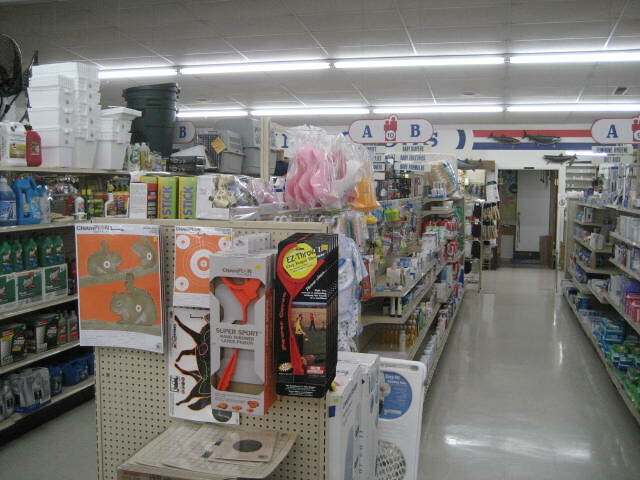A brightly lit aisle (aisle 10) of a store, illuminated by white lights, featuring shelves stocked with various products. The aisle floor is lined with linoleum, and both sides are labeled with identifiers "A," "A," and "B." The ceiling is adorned with tiles, and white lights also prominently shine above the firewood section. Products on the shelves include a mix of containers, cans, and plastic-wrapped items. In the foreground, there are sporting goods, such as targets depicting rabbits and squirrels, a slingshot packaged in a red 'claw' design, and more. Two individuals, dressed in red, are visible near the aisle number sign. Towards the back, a shelf holds bottles and containers in black and white, leading to what seems to be a crate. The background features a door, with a wall display of three plastic sharks, accented by red, white, and blue stripes.